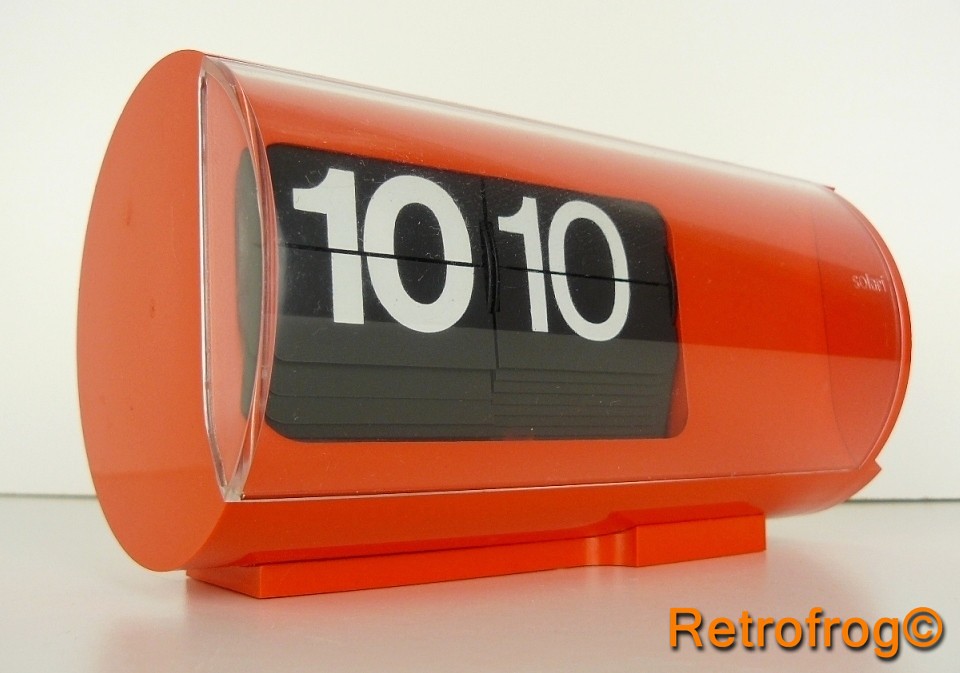A highly stylized alarm clock from the 1970s, characterized by its vibrant orange hue, stands prominently in the scene. The clock is almost cylindrical, with the open end facing the left, while the right end remains out of view. It perches on an equally orange base, creating a seamless and bold aesthetic. The front of the cylinder features a clear plastic cover, encompassing roughly 20% of the clock's surface. Beneath this transparent shield lies a flip numerical display, presenting a striking contrast with its black background and crisp white digits, currently showing the time as "10:10." In the lower right-hand corner of the clock’s face, the phrase "retro frog" is delicately inscribed in a light orange color, accompanied by a small copyright symbol, paying homage to the era's design trademark.